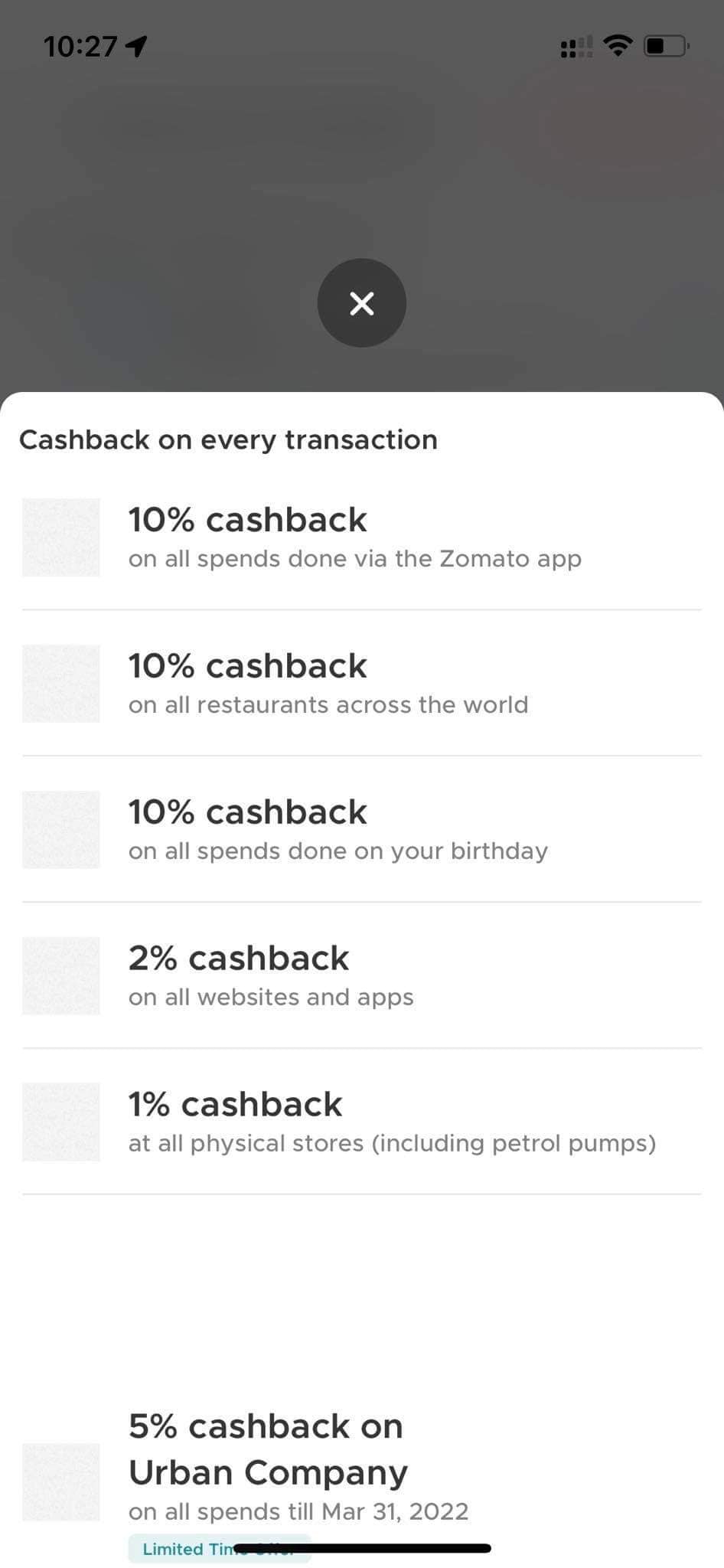The image features a promotional flyer with a predominantly white background. At the top, the text "1027 for Tom" is displayed, accompanied by a small gray circle with an 'X' inside it. Below this header, the flyer outlines cashback offers available through the Zoom Motto app:

1. A gray rectangular icon introduces a section that details a **10% cashback** on all expenditures made via the Zoom Motto app.
2. Another gray rectangular icon highlights a **10% cashback** on all restaurant transactions globally.
3. A further section, marked by a gray squared icon, features a **10% cashback** on all spends made on your birthday.
4. Another benefit listed with a gray icon offers a **2% cashback** on all online purchases through websites and apps.
5. Additionally, a gray squared icon details a **1% cashback** on transactions at all physical stores, including petrol pumps, as noted in parentheses.
6. There is also a specific mention of a **5% cashback** on all services booked through Urban Company.

The flyer specifies that these offers are valid on all spends till March 31, 2022, emphasizing that this is a limited-time opportunity. Towards the bottom, a black bar appears to strike through the remainder of some text, suggesting exclusions or terms that are not fully visible. The text and offers are rendered in blue, set against a light blue rectangular background, drawing attention to the promotional details.